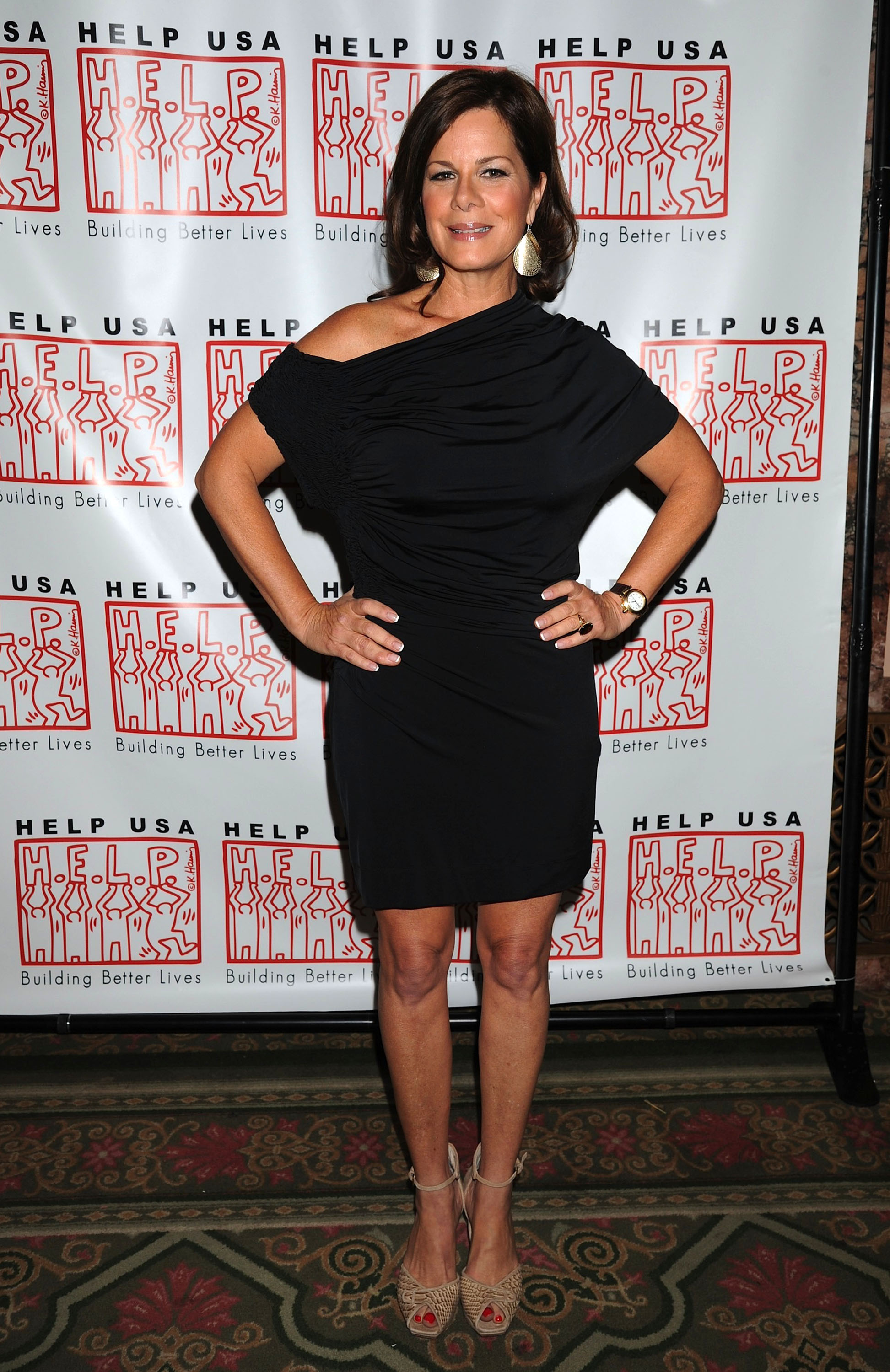In the image, an actress in her mid-40s is confidently standing in front of a banner that reads "Help USA Building Better Lives," which features a red rectangle with stick figures holding up the word "HELP." She is dressed in a short black cowl neck dress that is form-fitting on the bottom and slightly loose on the top, with one shoulder exposed. She has tanned skin and her red-painted toenails peek through her beige pumps. Her nails are well-manicured and she wears a black watch and large, shiny earrings that blend silver and gold tones. Her hair falls to her shoulders. The floral-design carpet beneath her adds a subtle decorative touch to the overall scene. She is the lead actress in the show "What About Todd," portraying the mother, and her confident stance—with hands on her hips—further enhances her commanding presence.